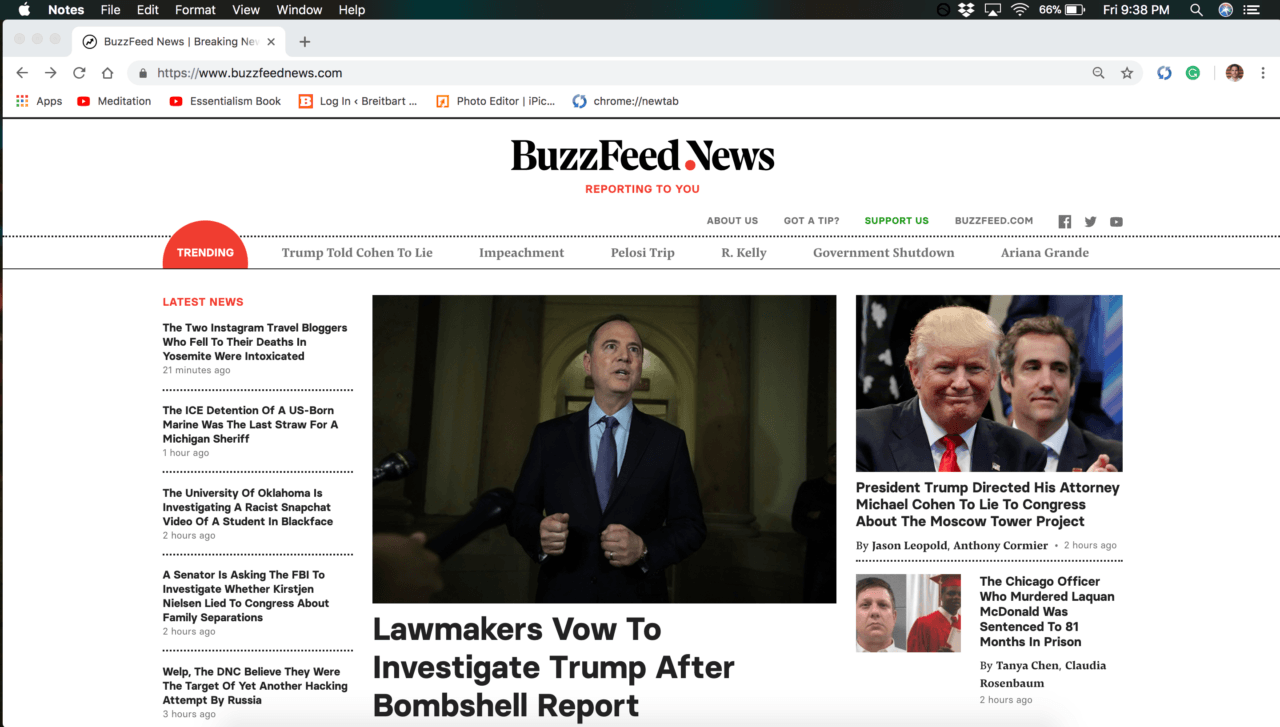This detailed caption describes a screenshot of a BuzzFeed News website viewed on what appears to be an iPad. The screen displays a typical white background with the navigation bar visible at the top, indicating the website's URL: https://www.buzzfeednews.com. Above the navigation bar, there is a black bar where the interface elements are displayed, featuring the Apple logo on the far left, followed by menu options like Notes, File, a partially obscured option, Format, View, Window, and Help. On the far right, icons for Dropbox, Wi-Fi, and battery status are visible.

Centered just below the navigation bar, the BuzzFeed News logo is prominently displayed with the tagline "Reporting to You" in red. Beneath this are various site navigation links, including "About Us," "Got a Tip," "Support Us," and "BuzzFeed.com," alongside social media icons for Facebook, Twitter, and Instagram. 

Further down, a red semicircle labeled "Trending" stands out on the left side, highlighting hot topics such as "Trump Told Cohen to Lie," "Impeachment," "Pelosi Trip," "R. Kelly," "Government Shutdown," and "Ariana Grande." Adjacent to the Trending section is the "Latest News" category, featuring five headlines. 

On the far right, a photograph of President Trump accompanies a headline that reads, "President Trump directed his attorney Michael Cohen to lie to Congress about the Moscow Tower project." Below this is a small thumbnail image of two individuals with the caption, "The Chicago officer who murdered Laquan McDonald was sentenced to 81 months in prison."

The central and most prominent image on the page is of a man in a dark suit with a blue shirt and blue tie. The headline beneath this image reads, "Lawmakers vow to investigate Trump after bombshell report."